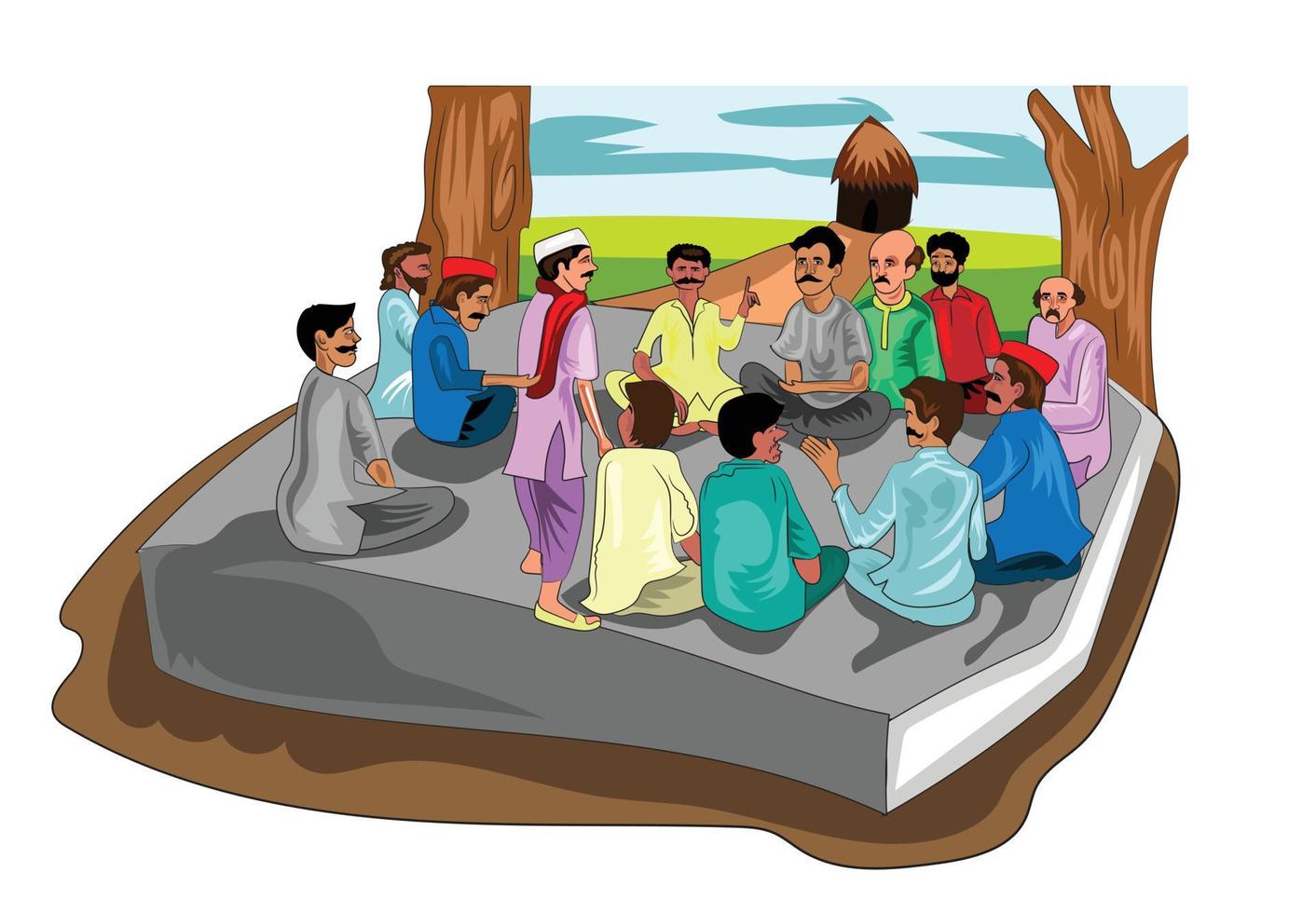This cartoonish image depicts a group of Middle Eastern men seated on a large rock or cement base. All the men sport short brown hair and mustaches, with some showing signs of balding. Three of the men are donning small caps. The men are dressed in outfits consisting of long, flowing shirts and matching pants, with at least one individual wearing flip-flops. One gentleman among them is also adorned with a scarf. The scene is set outdoors, flanked by two trees on either side, under a clear blue sky. Green grass surrounds the area, and a dirt or gravel path leads to a hut in the background, which has a natural roof. The overall vibe of the image is relaxed, capturing a moment of calm and camaraderie among the men.